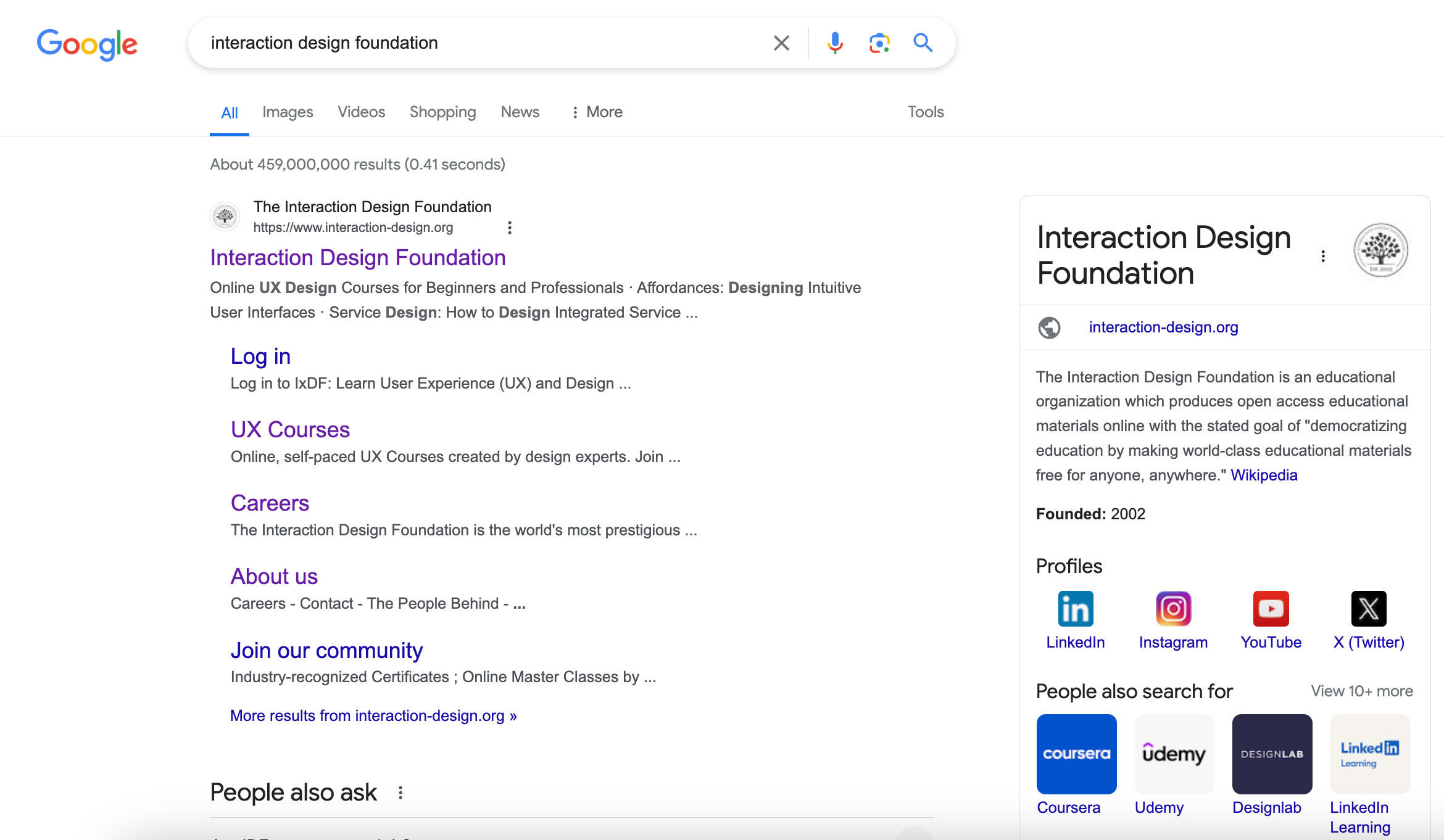Screenshot of Google search results for "Interaction Design Foundation." The search query is visible in the search bar at the top. Prominently, on the right side, there is an information panel detailing the organization. This panel includes the heading "Interaction Design Foundation," followed by the organization's official website link. A concise description under the heading reads: "The Interaction Design Foundation is an educational organization which produces open access educational materials online with the mission of democratizing education by making world-class educational materials free for anyone, anywhere." Below this description, there is a Wikipedia link displayed in blue, indicating the foundation was established in 2002.